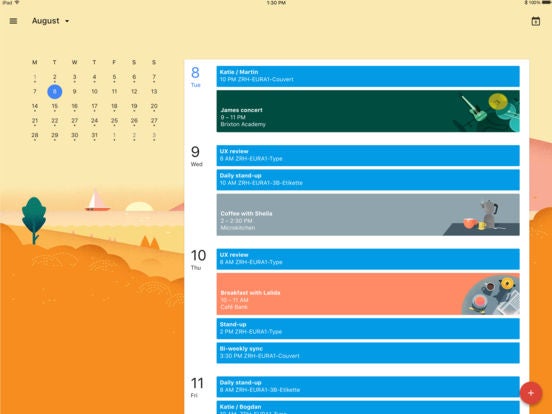The image appears to be a screenshot of an iPad displaying a calendar interface for the month of August. At the top left corner, it prominently displays the term "iPad" along with the current time, which reads either 1:30 or 1:36 p.m. On the top right, there is a battery indicator.

In the foreground, the calendar is opened to the week containing August 8th through August 11th. The selected date is August 8th. Various appointments are visible on these days, color-coded for easy differentiation: blue, dark green, blue again, gray, and orange.

The background features a scenic illustration of orange mountains beneath a sky. Additionally, a slight yellow-tinted ocean with a visible sailboat can be seen. There is a single green tree present, adding to the picturesque landscape. In the upper left of the calendar interface, a smaller version of the full month of August calendar is displayed, showing all the days of the month for quick reference.